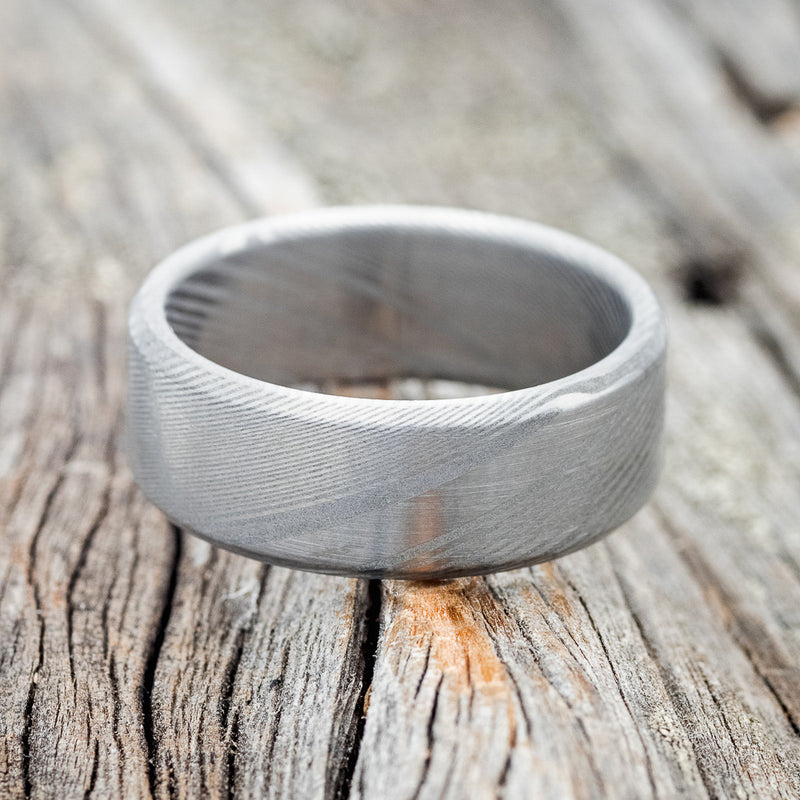The photograph showcases a substantial, brushed silver ring, likely a male wedding band, prominently positioned on a weathered, rustic wooden bench that resembles a well-maintained pub bench. The ring, which fills about one-third of the image, features an intricate engraved pattern with diagonal stripes, adding texture and depth to its thick band. The wood beneath it is light-colored and displays numerous cracks and a missing knot, emphasizing its weathered appearance. The background gradually blurs out, highlighting the texture and wear of the old, cracked wood in the foreground. The entire composition comprises various shades of brown from the bench and the striking silver of the ring, creating a visually appealing contrast. This detailed presentation suggests that this might be a professional photograph aimed at showcasing the ring for an online listing, possibly on platforms like Etsy.